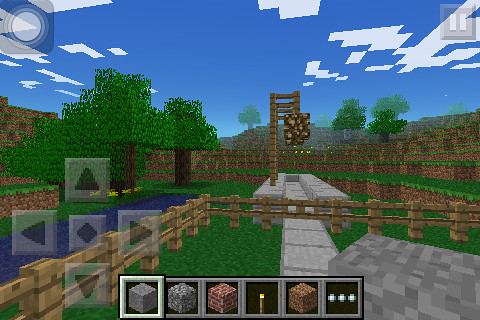The image is a screenshot from a Minecraft game, showing a first-person perspective of a player character. In the bottom right corner, the player is holding a gray smooth stone block. The top of the image features a bright blue sky with a few scattered blocky white clouds. Directly ahead, there is a wooden fence with a gated stone pathway extending into the distance. Lining the pathway, tall wooden poles with light fixtures can be seen. To the left of the pathway, there is a serene, dark blue pond bordered by brown dirt and vibrant green trees. Beyond the immediate scene, hilly terrain stretches out into the horizon.